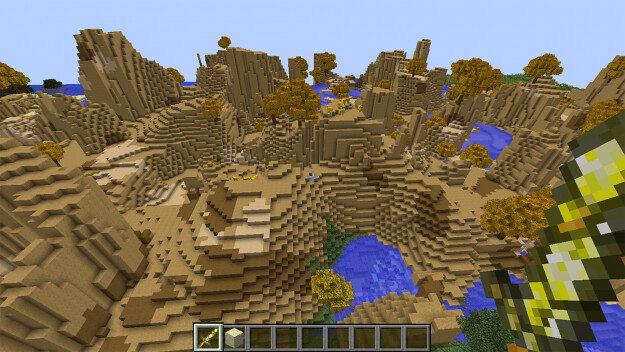This computer-generated image depicts a stylized landscape with a blocky, pixelated appearance. The landscape features medium, dark, and light brown stacks that form a topographical map-like structure. Scattered throughout this terrain are several dark blue pools of water. Across the top of the image, light blue hues simulate the sky.

In the center bottom, a grid of blocks is visible. The first block on the left contains a yellow sword, while the adjacent block holds a box; the remaining blocks are empty. On the right side of the image, various stacked colors include black, yellow, and white, adding to the diverse texture of the scene.

Additionally, the landscape includes green patches and yellow flowers with green leaves, possibly indicating vegetation. There are also hints of yellow that might represent trees. In the distance on the right side, green shapes suggest hills, while black formations on the left hint at rocky outcrops. This intricate composition creates a detailed, topographical representation of a pixelated terrain.